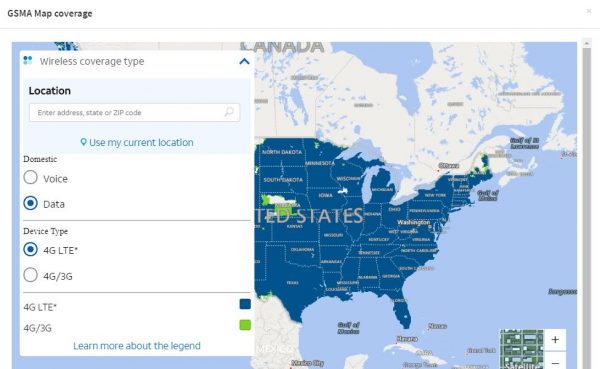The image appears to be of a website interface focused on displaying mobile service coverage in the United States. At the top left corner, there is prominently displayed black text that reads "GSMA Coverage Map." Below this header, there is a partially visible map of the United States, colored in blue, extending from Texas to North Dakota and South Dakota. The map also shows bordering regions such as Canada and Mexico, as well as adjacent oceans, with state names labeled in gray text.

To the left of the map, there is an informational box with the title "Wireless Coverage Type" in gray text at the top. Below this, bold black text reads "Location," accompanied by input fields where users can enter their address, state, or zip code. Additionally, there is a blue text link that says "Use My Current Location."

Further down, there is the option to select between "Domestic" categories, labeled with smaller black text, which includes choices for "Voice" or "Data." In the example, the "Data" option is selected. The user can also choose the type of device, with "4G LTE" selected instead of "4G/3G."

At the bottom of the box, there are labels indicating "4G LTE" with a blue dot and "4G/3G" with a green dot. The interface concludes with an option in blue text that reads "Learn More About the Legend."